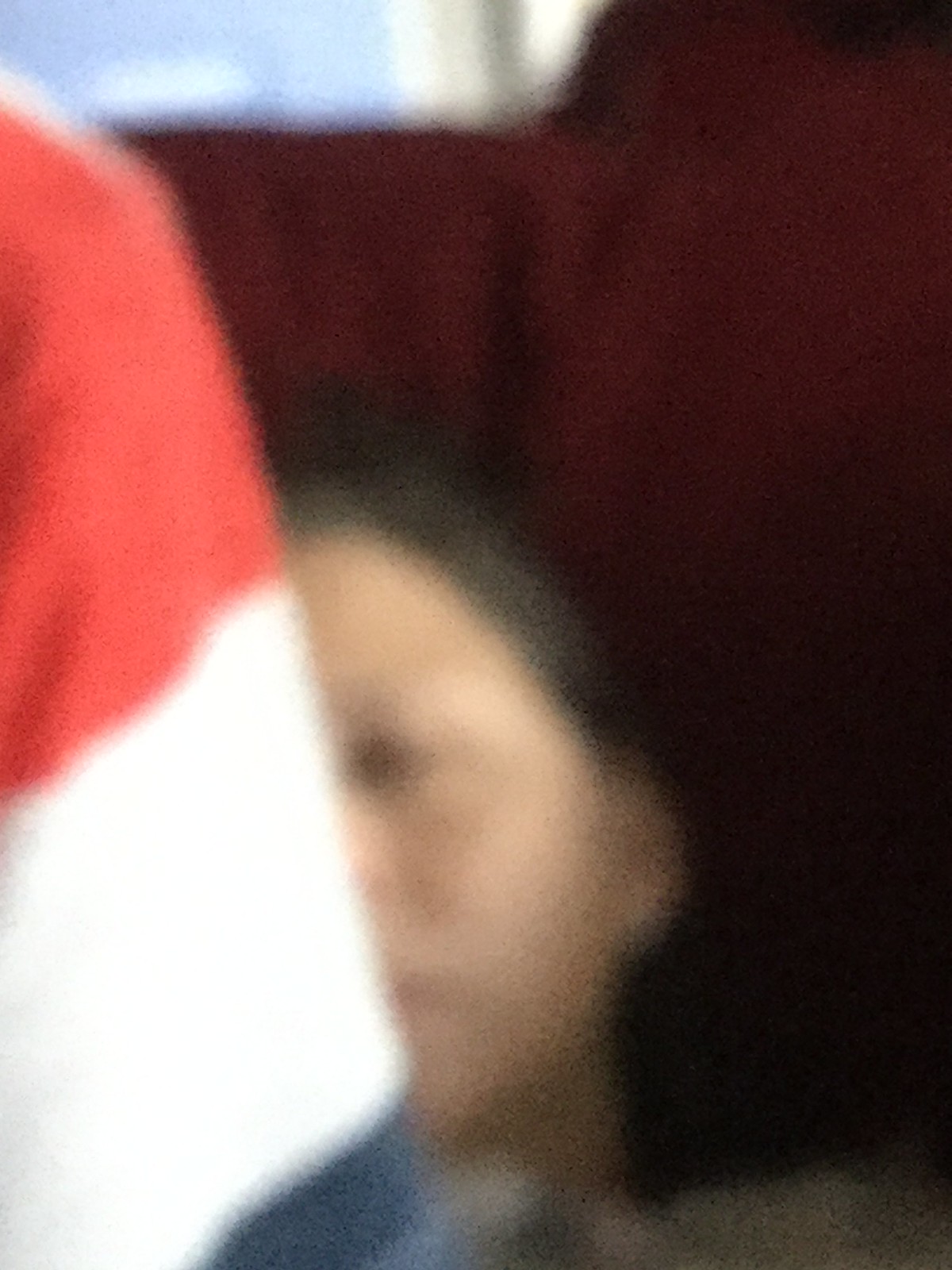The image is a very blurry and pixelated photo featuring the left side of a person's face, which is partially obscured by someone's shoulder and sleeve. The person in the foreground is wearing a shirt with a red, white, and blue striped pattern. The individual whose face is visible appears to have dark, possibly black hair with hints of gray, which might be pulled back. The visible features include one eye, half of the nose, and part of the lips, suggesting the person could be Hispanic. The background consists of a reddish-burgundy fabric, likely a sheet, blanket, or pillow. Additionally, at the top of the picture, there is a visible area that could be a phone screen or a console device resting on the bed, along with some shiny white and beige elements that might be part of the surrounding environment.